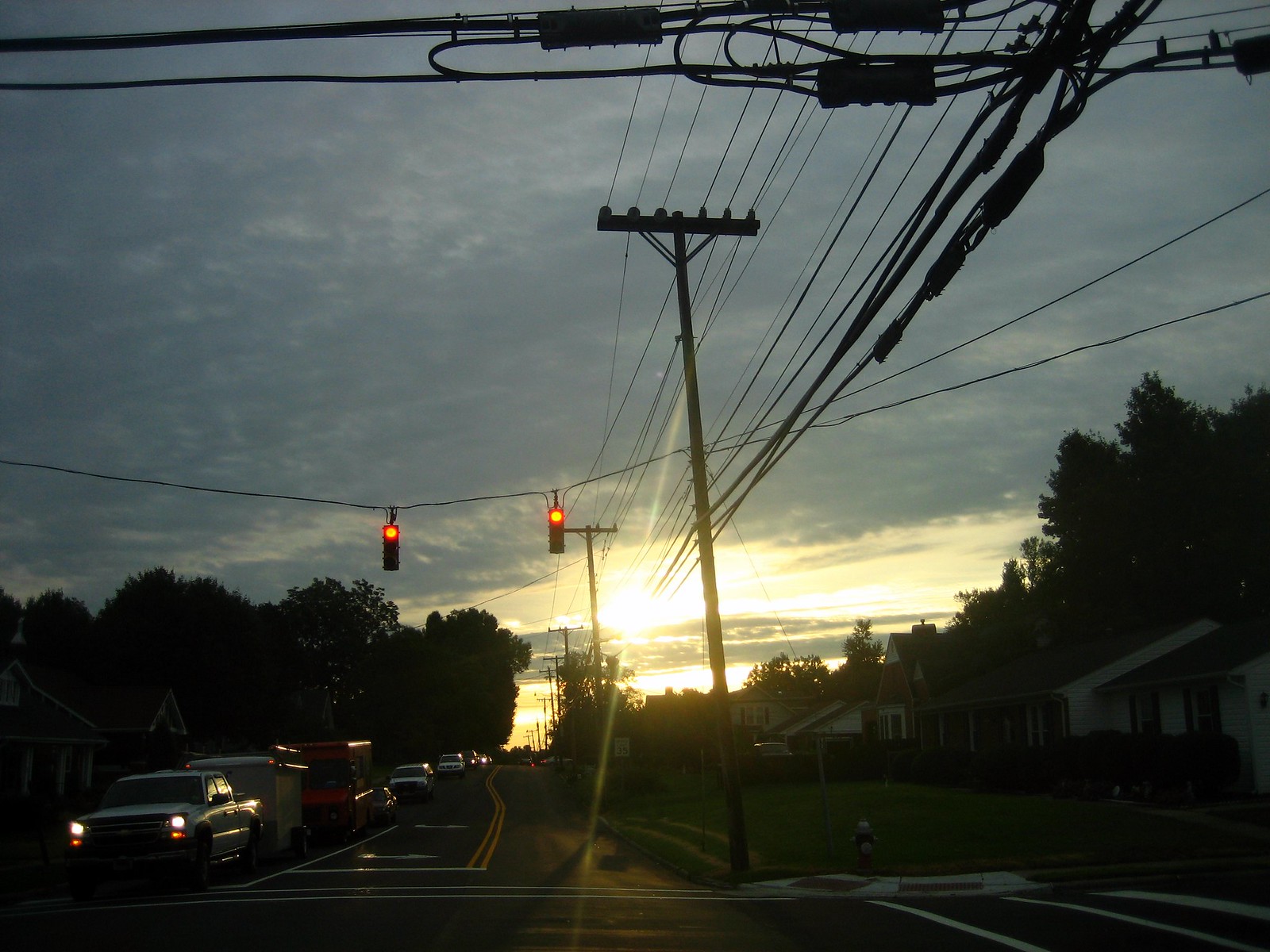This first-person perspective image captures the serene moment of a sunset as seen through a car windshield or possibly from a camera extending out of the window. The setting sun, partially obscured by scattered clouds, bathes the sky in vibrant hues of orange and yellow, casting a warm glow across the scene. The car from which the photo is taken is stopped at a T-intersection, with the traffic light showing an orangey-red indication. The scene unfolds from the right-hand lane, poised to move straight ahead, while on the left-hand lane, a long line of cars extends beyond the picture's frame, waiting their turn. Overhead, an array of power lines and poles on the right-hand side stretches into the distance, accentuating the depth of the roadway. The combination of the glowing sunset, the lined-up vehicles, and the intricate play of light and shadow creates a captivating moment of everyday life paused in twilight.